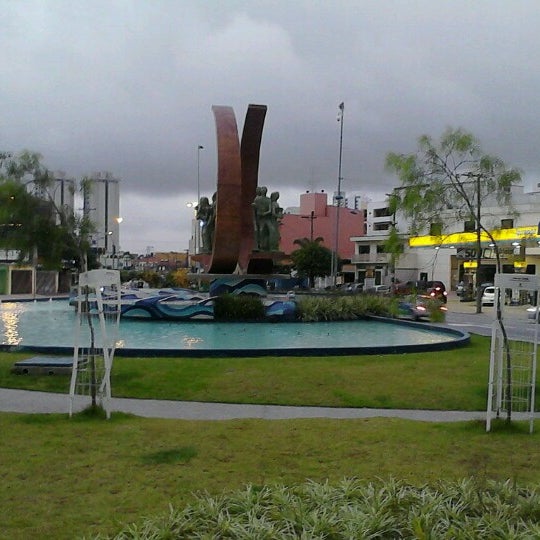The image captures a section of a city, focusing on a large decorative fountain in the center of a shopping district. The fountain is a shallow pool with a tall artistic sculpture at its core, composed of two red semicircles extending upwards amidst wavy blue stone elements. Encircling the semicircles are statues of people made of metal, forming a striking monument. The pool's edge is marked by a black border, and there is a sidewalk between the pool and the foreground of the image.

Surrounding the fountain, there are scattered bushes, a path that meanders through grassy areas, and two trees supported by some kind of structures. In the immediate foreground, low bushes are visible. To the right of the fountain, a white building with a yellow awning stands out, and next to it, a pink multi-storied building can be seen. Far to the left in the distance, two skyscrapers emerge against an extremely cloudy and dark sky, adding to the dramatic atmosphere.

Additionally, some white device, possibly a netting, is present, though its exact function is unclear. Sparse water droplets are visible towards the right side of the image, suggesting it might be raining, given the overcast sky. The detailed architectural and natural elements indicate that this is a location intended for people to visit and enjoy.